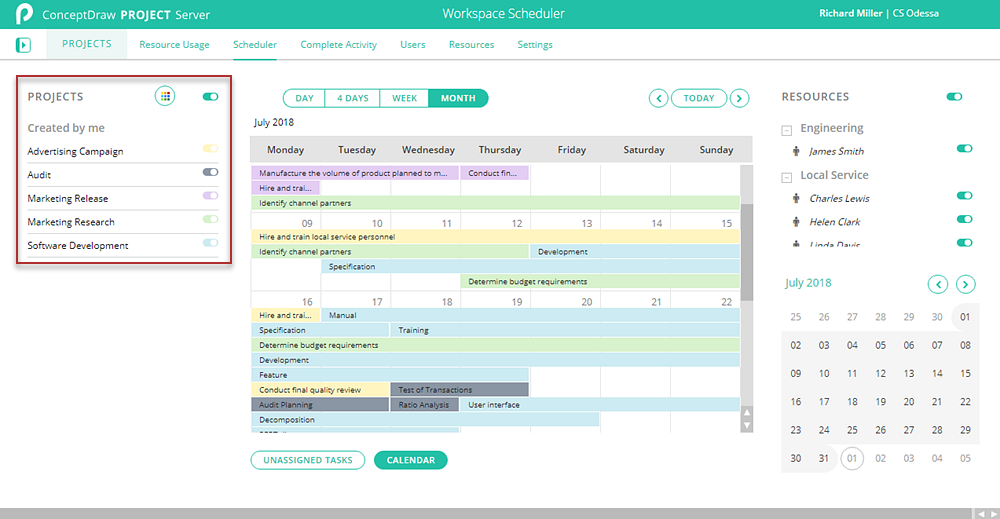The image displays a screenshot of a project management software interface. At the top, a green bar features white text stating "ConceptDraw Project Server." In the center, the screen reads "Workspace Scheduler," while the top right corner shows the user information "Richard Miller, CSO, Odesso."

Below this, a white area features a green menu with options titled "Projects, Resource Usage, Scheduler, Complete Activity, Users, Resources, Settings." On the left side, within a red-bordered box labeled "Projects," there is a subheading "Created By Me." This section lists various project options such as "Advertising Campaign, Audit, Marketing Release, Marketing Research, Software Development," each accompanied by color-coded buttons.

To the right, a calendar interface is displayed. The top of the calendar offers viewing options labeled "Day, Four Days, Week, Month" and shows the days of the week from Monday to Sunday. Various tasks are highlighted in different colors; for example, "Identify Channel Partners" is marked in green, while "Development" and "Specification" are marked in blue.

Below the calendar, there are buttons for "Unassigned Tasks" and "Calendar," with the full calendar for July 2018 prominently shown. Additionally, the right-hand sidebar contains sections titled "Resources, Engineering, and Local Service."